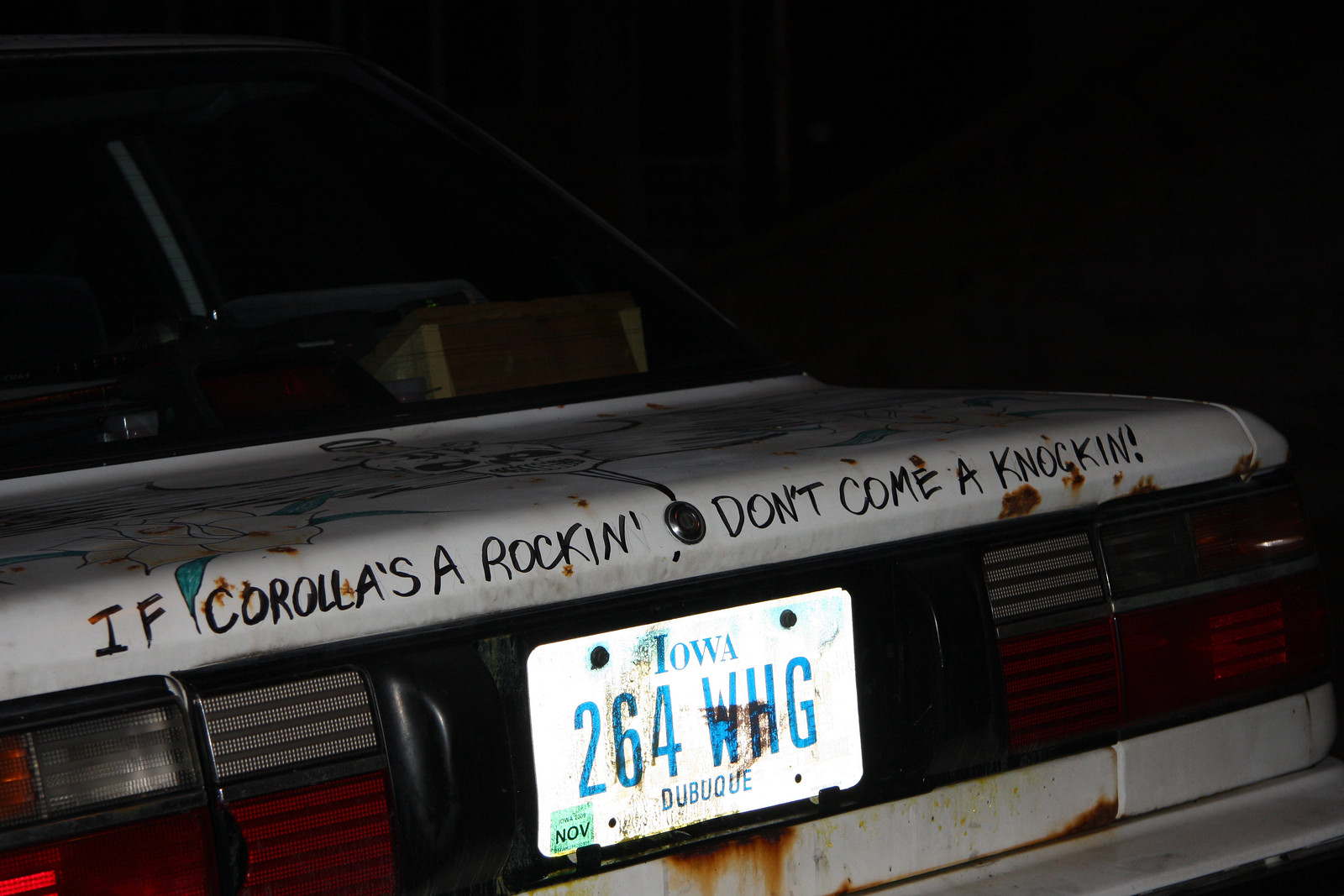This close-up image of the back of a white, older Toyota Corolla, taken at night, shows detailed wear and tear, including noticeable rust spots and rough patches. The back windshield is visible, and the trunk features a distinctive artwork, including a painted skull and other designs, though they are somewhat faded and hard to discern. Centered around the keyhole, there is a playful message in black letters: "If Corollas are a-rockin', don't come a-knockin'." The car has an Iowa license plate, predominantly white with a blue top reading "Iowa," followed by the plate number "264WHG" and "Dubuque" beneath it. A green November sticker is affixed to the bottom left corner of the plate. The background of the image is completely black, emphasizing that it was taken at night.